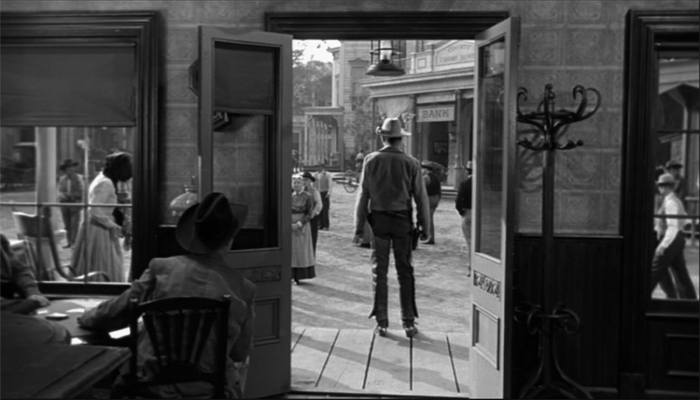This black-and-white photograph captures the quintessential old Western scene, likely taken inside a saloon. The focus is on a cowboy sitting on a black chair to the left of the image, donning a dark cowboy hat and jacket, and possibly engaged in a game of poker as his gaze is drawn toward the scene outside. A table is positioned before him, adding to the saloon atmosphere. Directly to his left, an arm of another individual rests on the table, suggesting he's not alone.

The saloon features windows and an open door that frames the outdoor setting. Outside, standing on a wooden deck porch, another cowboy in a light hat gazes outward. He is equipped with firearms on his hips, clad in leather pants and black boots, embodying the rugged lawman or gunslinger archetype. The porch overlooks a bustling yard where several figures in Western attire, including more cowboys and a lady in a colonial dress with a cap, move about.

In the distance, a building marked "Bank" stands prominently, contributing to the evocative setting. The right side of the saloon accommodates a coat rack near another window, amplifying the sense of a lived-in, period-specific environment. Through the open doors and windows, various elements like a large pillar, more buildings, and a cartwheel can be spotted, all anchoring the image firmly in a bygone era of the Wild West.